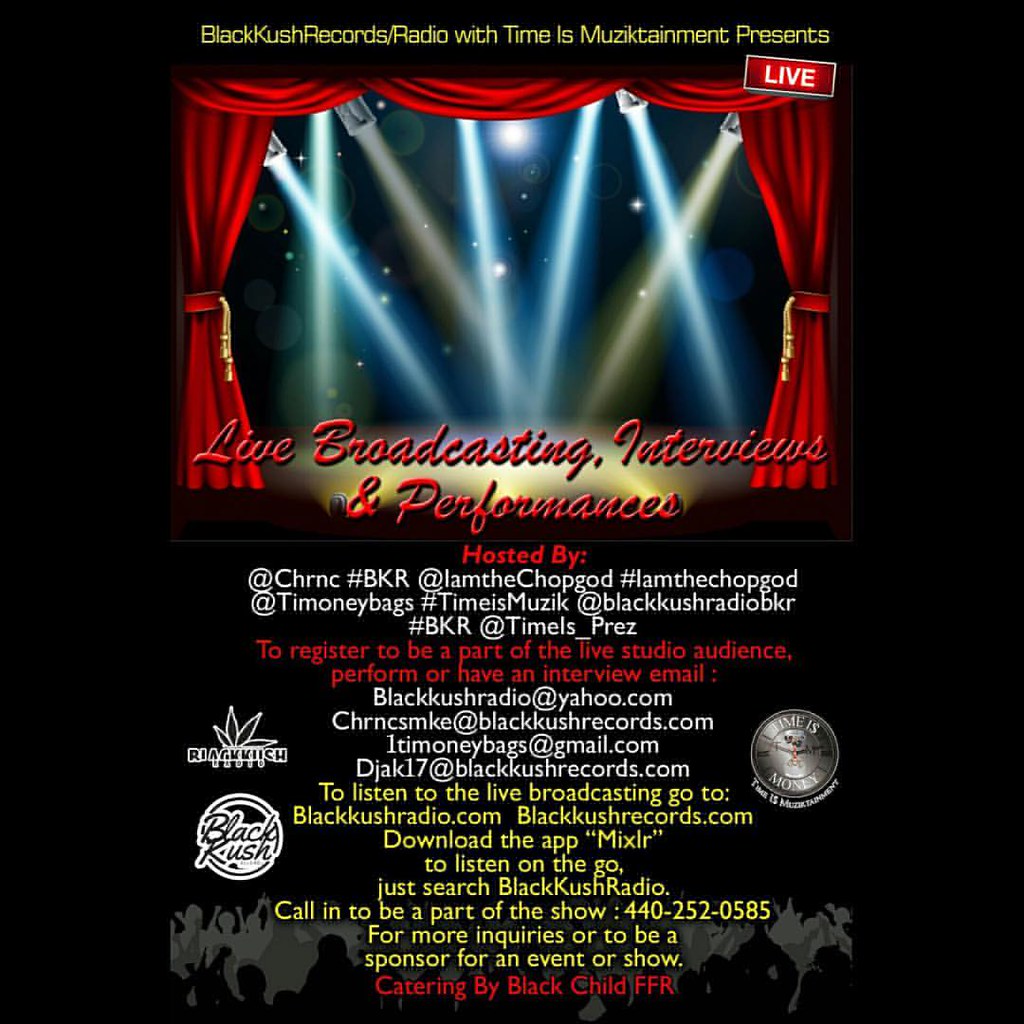The image appears to be a detailed computer-generated flyer featuring a predominantly black background. At the very top, in bold yellow letters, it reads: "Black Kush Records Radio With Time is Music Segment Presents." Beneath this heading, a picture of a stage adorned with red curtains and illuminated by spotlights is prominently featured. In the upper right-hand corner of the image, the word "Live" is displayed.

In elegant red cursive text, it announces: "Live Broadcasting Interviews and Performances Hosted By." Below this announcement, a list of hosts is provided, including Chronic BKR, I Am the Chop God, Ti Money Bags, Time is Music, Black Cush Radio, BKR Timeless, and Prez. Various email addresses are listed for those interested in registering to be part of the live studio audience, perform, or be interviewed. Additional contact options include a phone number (440-252-0585) for call-ins and inquiries.

Further details in white text direct viewers to listen to the live broadcast via multiple platforms: blackkushradio.com, blackkushrecords.com, or by downloading the Mixlr app and searching for Black Kush Radio. Twitter and Instagram handles are also incorporated, offering social media engagement. At the bottom, in red text, it mentions that catering is provided by Black Child FFR. Flanking the overall design are various white logos, adding a professional touch to the flyer.